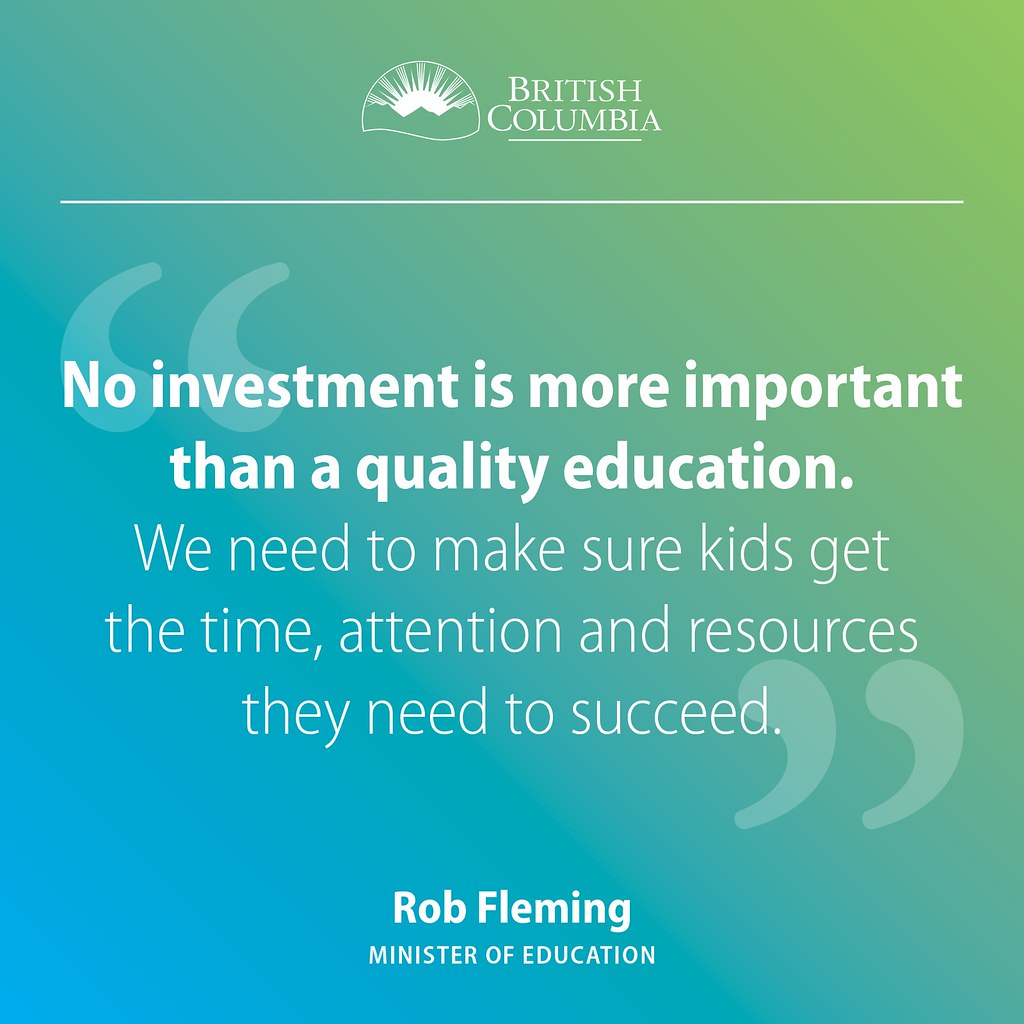The image features a large square design split into two main colors: the lower half is blue, and the upper right half is green. At the very top is a logo of a sun outlined in white with green shading beneath, representing mountains, next to the text "BRITISH COLUMBIA" in all caps, white letters, underlined. Below this header, a horizontal line separates it from the main body of text. The centered text reads: "NO INVESTMENT IS MORE IMPORTANT THAN A QUALITY EDUCATION" in bold white letters. Directly underneath, also centered but in non-bold white letters, it states, "We need to make sure kids get the time, attention, and resources they need to succeed." At the bottom, the name "ROB FLEMING" appears in bold white letters, followed by "MINISTER OF EDUCATION" in all caps, non-bold white letters. The overall style suggests a motivational or promotional message possibly related to an education initiative from Rob Fleming in his role as British Columbia's Minister of Education.